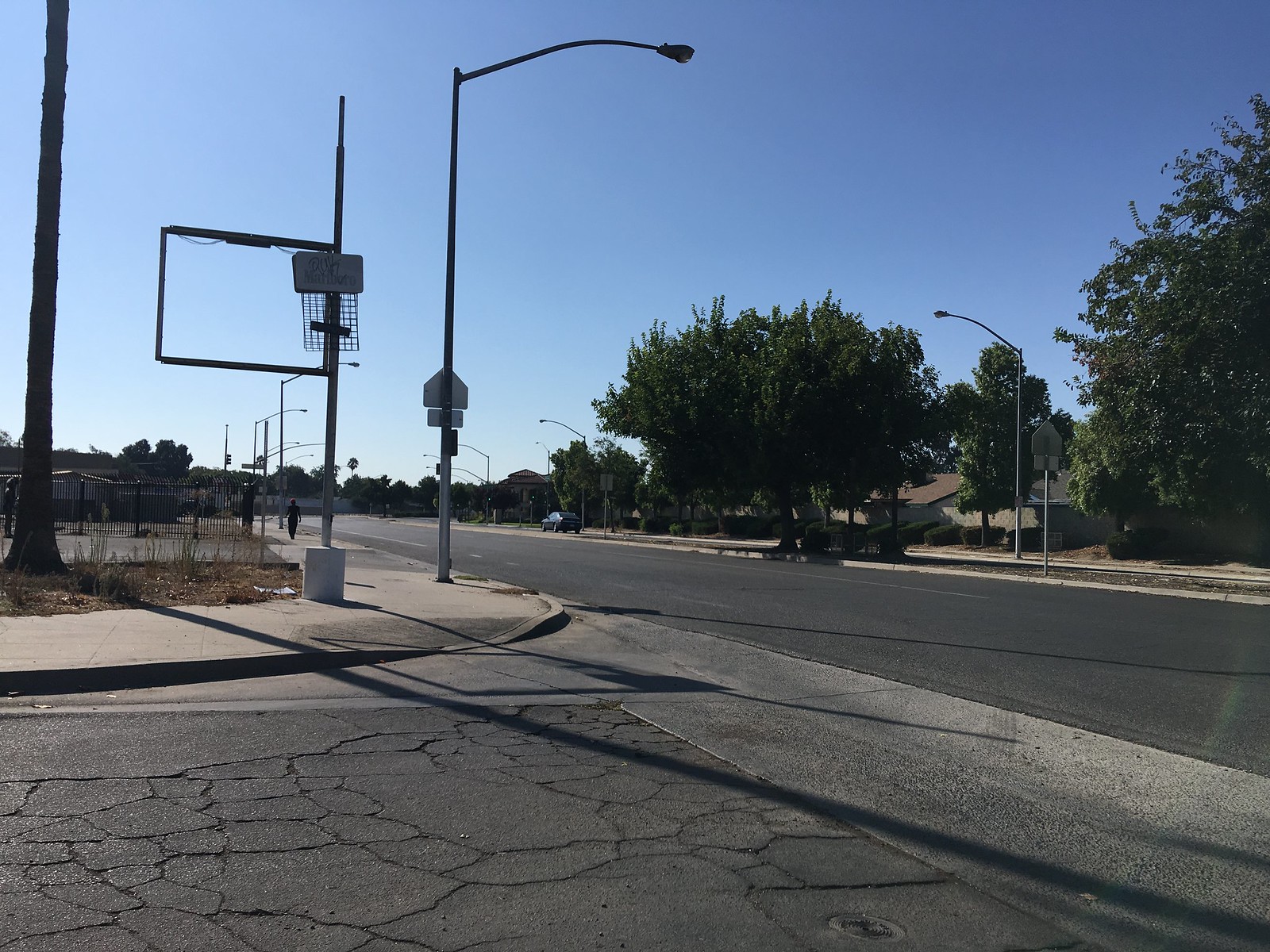This photograph captures a street corner in a seemingly deserted area. The prominent feature is a major highway running across the foreground, with an alleyway or side street emerging and merging onto this highway. The macadam on this side street is extensively damaged, resembling a jigsaw puzzle with numerous pieces fragmented but still on the ground, indicating it is in dire need of repair.

The street signs present an intriguing detail: the name "Hatboro" (spelled H-A-T-T-B-O-R-O), is visibly crossed out with "Philly" written above it. Among the street furniture, there’s a notable grid-like structure mounted on one pole and the reverse sides of some light post signs are visible.

Further down the street, a large gate is visible, suggesting the presence of businesses or a parking lot beyond it. One person is seen walking on the street, adding a human element to the scene. Across the street, a single car is parked, and a cluster of trees can be seen. However, this side of the street lacks greenery except for what appears to be a tall, leafless pole-like tree without branches, contributing to the desolate ambiance of the area.